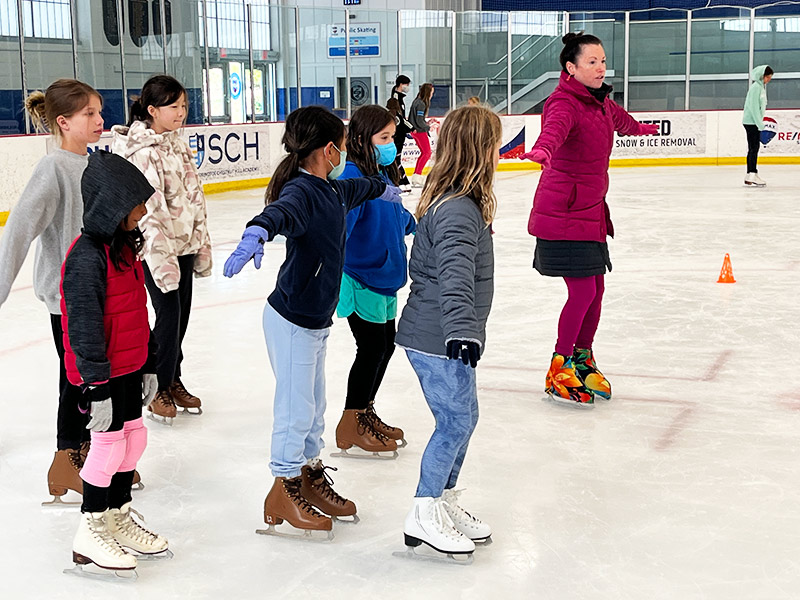The photograph captures an ice skating lesson inside an enclosed rink with glass walls, adorned with signage including "SCH Snow and Ice Removal" and "REMAX." In the foreground, six children, dressed warmly for the cold, stand on the ice with white or brown skates, mimicking their instructor. The instructor, a woman with dark black-brown hair, is wearing a burgundy jacket, a black skirt, and burgundy leggings with floral-patterned skates featuring orange flowers and green leaves. She has her arms outstretched, demonstrating a balanced stance with bent knees, which the children imitate intently. In the background, three other skaters participate in what seems to be a continuation of the lesson.